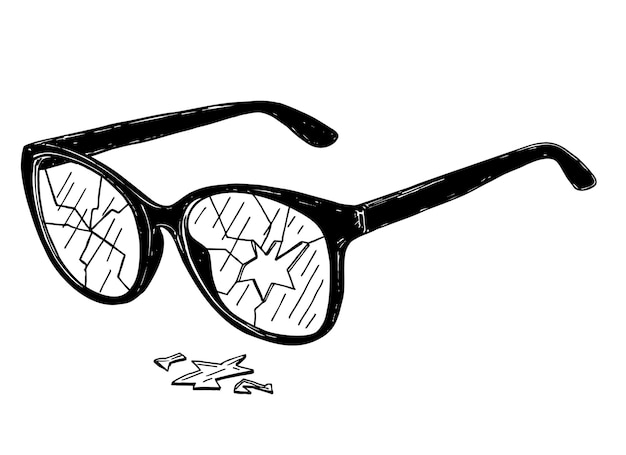The image showcases an artistic, black ink drawing of a pair of eyeglasses set against a pure white background. The glasses feature a black frame with black arms, oriented so that the corner of the left eye is closest to the viewer. Both lenses are shattered, with numerous jagged cracks, and a small, distinct piece of glass missing from the left lens. This broken piece of glass is depicted resting on the surface in front of the glasses. The scene is minimalistic, devoid of any text, numbers, or additional objects, highlighting the stark contrast between the black glasses and the white backdrop. The overall clarity and brightness of the image emphasize the intricate details of the shattered lenses and the design's simplicity.